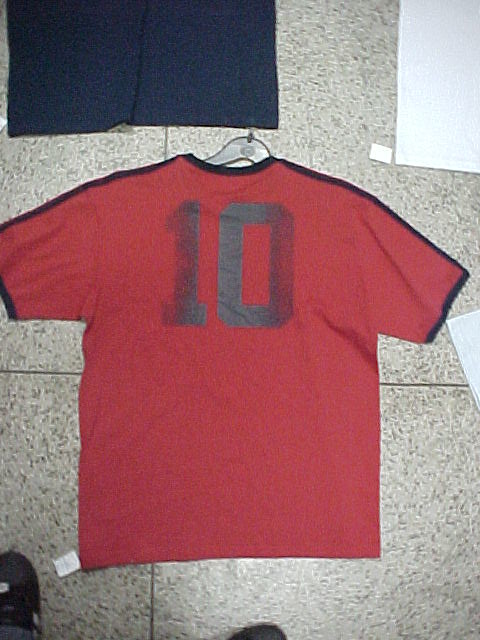This indoor color photograph, slightly out of focus and poorly taken, captures a red sports jersey laying flat on a grainy gray linoleum floor. The short-sleeved jersey, likely designed for a man, is predominantly dark red with black borders around the shoulders and sleeves. Displayed from the back, it prominently features a black number 10, which appears slightly faded along the edges. A black plastic clothes hanger supports the jersey, and a white tag is visible at the bottom left of the shirt. The floor below is segmented into square tiles. In the photo's lower left and lower edge, the tops of the photographer's shoes are visible. Additionally, the upper right corner shows part of another garment, presumably a blue-colored fabric with a tag, adding to the scene's cluttered appearance. The image is well-lit but captures the scene with a lack of precision.